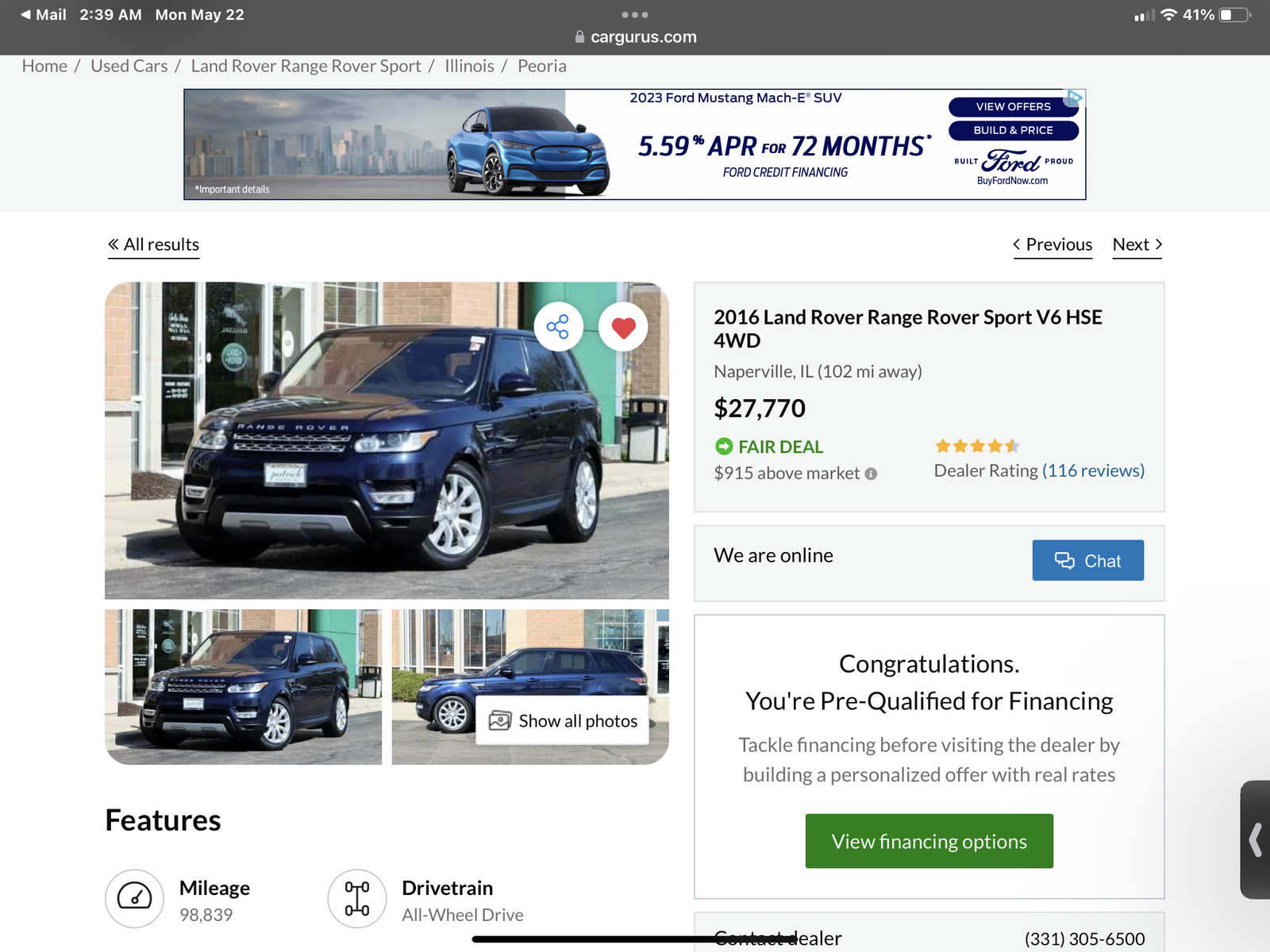This is a detailed screenshot of the CarGurus website as viewed on a mobile device. The page features a medium gray header that spans the top of the screen, displaying white text and icons in the top left, top right, and top center. Centrally positioned in this header are three horizontally aligned light gray dots. Beneath the header, a light gray lock icon is visible, followed by white text reading "cargurus.com."

Immediately below, a light gray subheader features dark gray text that reads: "Home / Used Cars / Land Rover Range Rover Sport / Illinois / Peoria." Below this section, an advertisement occupies a significant portion of the header area. 

This advertisement is prominent and wide, featuring a clear division between two notable visual elements. On the left side, there's a photograph depicting a dense skyline under a pale blue sky dotted with gray clouds, and an expanse of light gray asphalt in the foreground. White text on the bottom-left corner of the asphalt reads "Important details."

To the right of this cityscape image is a stark white background that highlights a shiny blue car angled slightly towards the camera. Overlaid on this white background is very large, italicized dark blue text that announces, "5.59% APR for 72 months*," with a smaller, all-caps blue subtext that reads, "FORD CREDIT FINANCING."

At the top of the advertisement, small blue text identifies the vehicle as a "2023 Ford Mustang Mach-E SUV." In the top right corner, the ad features two blue buttons stacked vertically, each with all-caps white text: "VIEW OFFERS" on the top button and "BUILD AND PRICE" on the bottom button. 

Overall, the image offers a comprehensive view of the CarGurus website layout and a prominent advertisement, seamlessly blending visual and textual content for a detailed user experience.